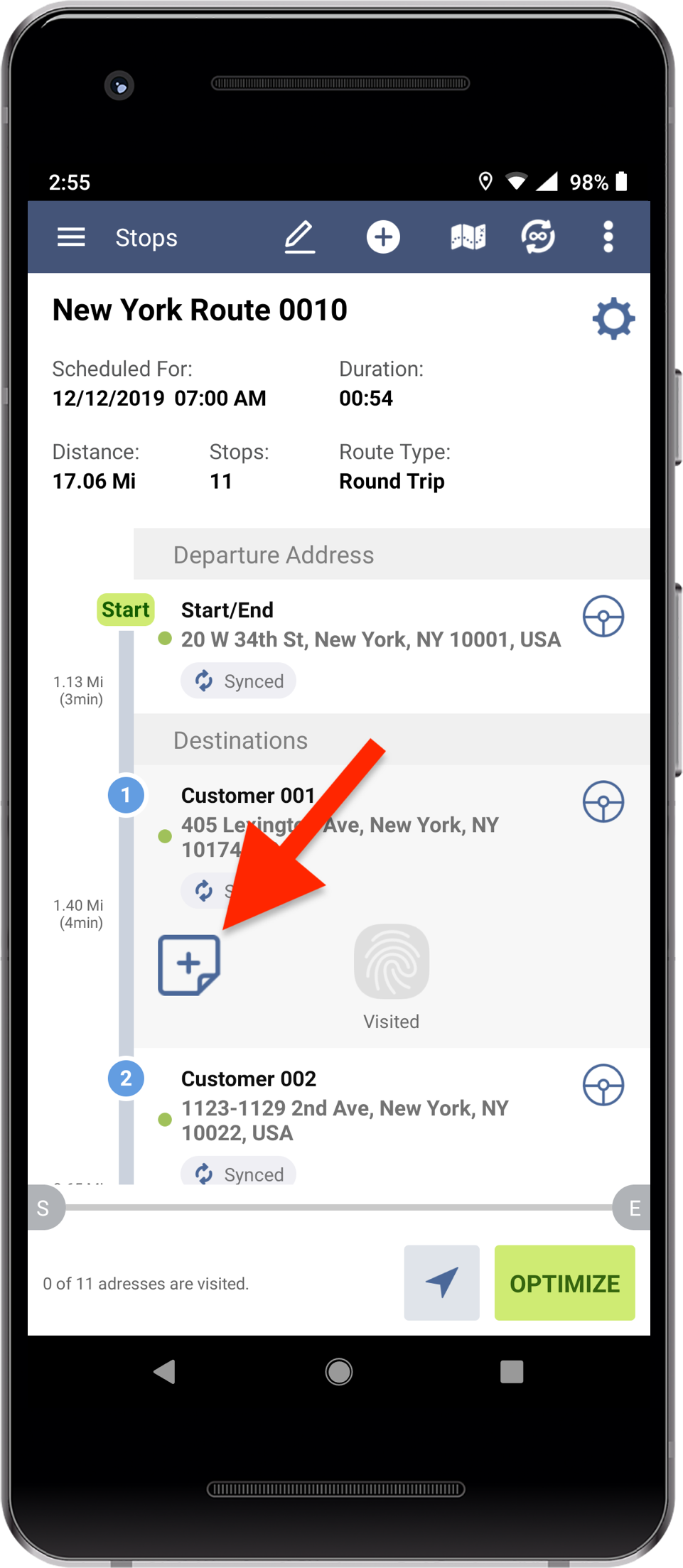This image is a screenshot depicting a graphical interface of a smartphone. The smartphone has black bezels surrounding its screen. At the top of the image, there is a black status bar. Displayed on the status bar in white font is the time "2:55," along with icons indicating that location sharing is on and showing the Wi-Fi and mobile signal strengths. The battery icon shows the device is at 98% charge.

Below the status bar is a blue navigation bar that reads "stops." On this bar, there are several icons: three vertical white lines, a pencil pressing down on a line, a circle with a plus sign inside it, a map, and a circle made of arrows with an infinity symbol in the center.

Further down, there is a white section that details a route. At the top of this section, it reads "New York route 0010," scheduled for "12/12/2019" at "7 AM." The route details include a duration of "00:54" (54 minutes), a distance of "17.06 miles," "11 stops," and indicate the route type as a "round trip."